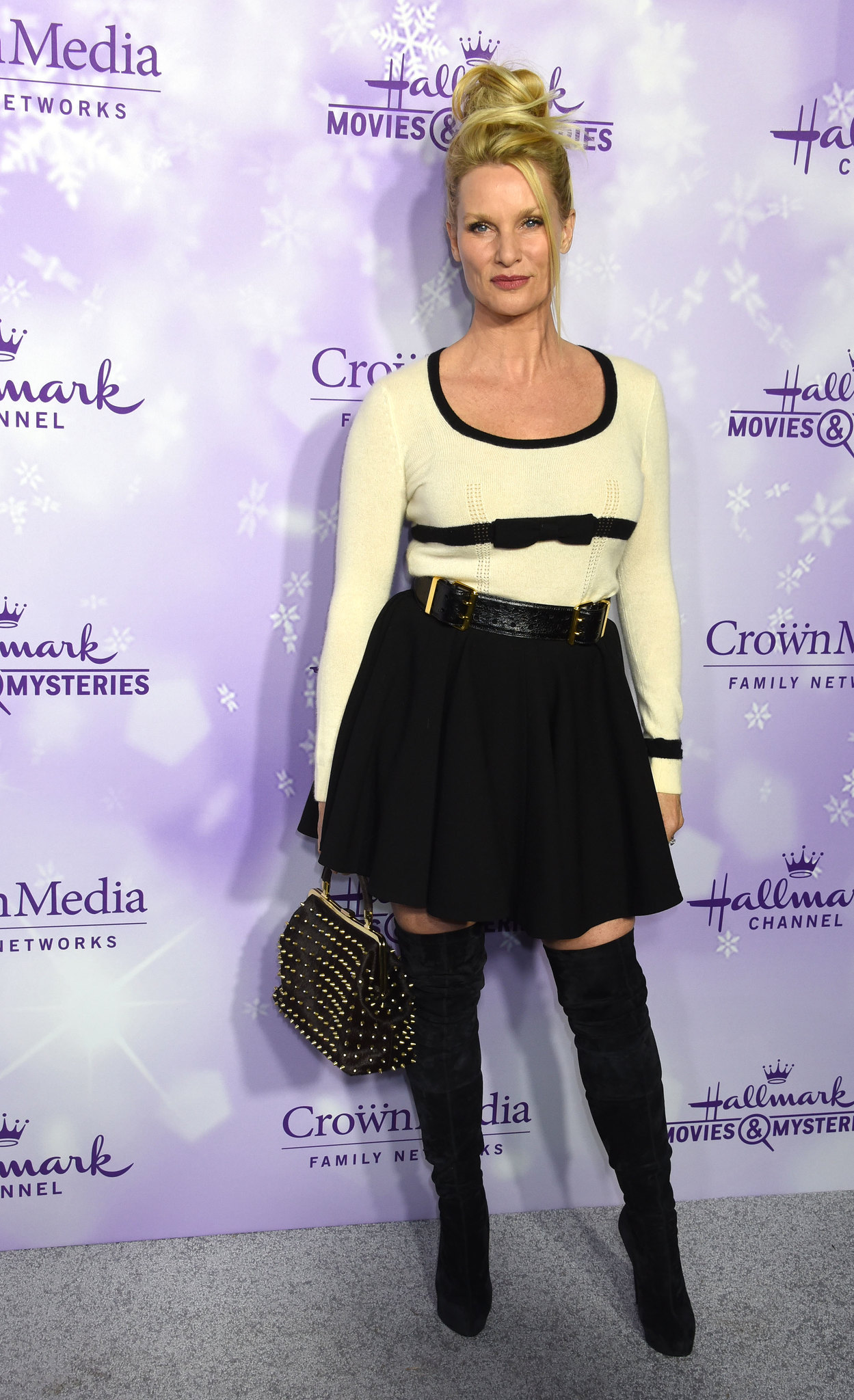The image features a woman in her late 30s with blonde hair styled in a high bun. She is facing the camera and has a confident expression. She is dressed in a white scoop neck sweater with black trim, black cuffs, and a distinctive black bow across the lower chest area. She pairs this with a pleated black mini skirt and a black and gold belt. Her accessories include a black handbag with gold trim, tall black boots that extend past her knees, and thigh-high socks. The background is a promotional backdrop with a repeated pattern of logos for Hallmark Movies and Mysteries and Crown Media Family Networks, featuring a lavender and white color scheme. The floor is covered in gray carpet.